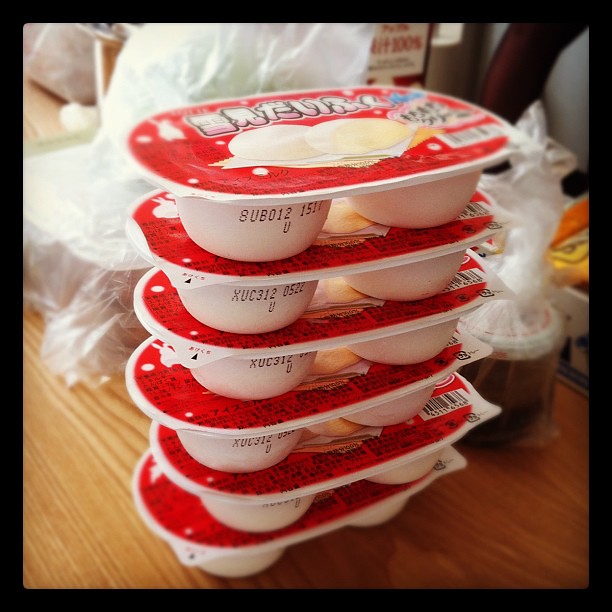This photograph showcases six vertically stacked snack packs, each consisting of a cylindrical, white plastic container divided into two sections, sealed with a red foil lid. The lid features Japanese writing in white with pink accents, alongside an image depicting two white, pillowy rice cakes, resembling mochi. One cup boasts legible alphanumeric codes, such as "8UB012" and partially obscured text "15," with variations like "XUC312052ZU" appearing on other visible cups. Positioned on a light brown table, the scene is cluttered with various items in clear plastic bags, including a glass container with a white and red lid and unidentified rectangular containers.